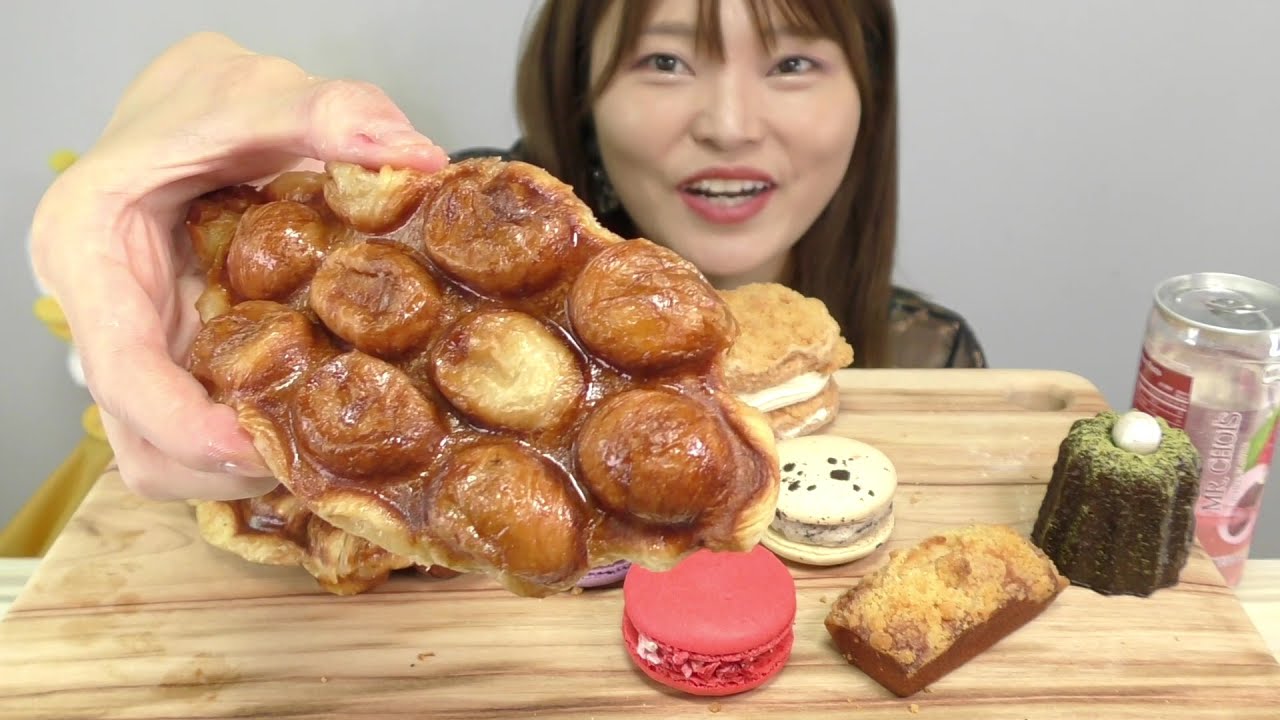In this photo, a smiling young woman of Asian descent with brown hair is showcasing an array of delectable treats on a wooden cutting board. Held prominently in her hand is a unique, glazed pastry resembling button shapes, possibly accented with butter, maple syrup, or honey. Surrounding her on the table are various other snacks including a crumb-topped coffee cake, a pink-hued hamburger-like dessert, a red cookie sandwich, a green dessert, and a piece of a chicken sandwich. An unopened silver and pink can of soda, likely labeled "Mr. Kohl's," is also visible amidst the assortment. The scene is set against a gray wall, with the woman slightly blurred in the background, highlighting the diverse range of sweets and treats she intends to present, possibly for a YouTube cooking video.